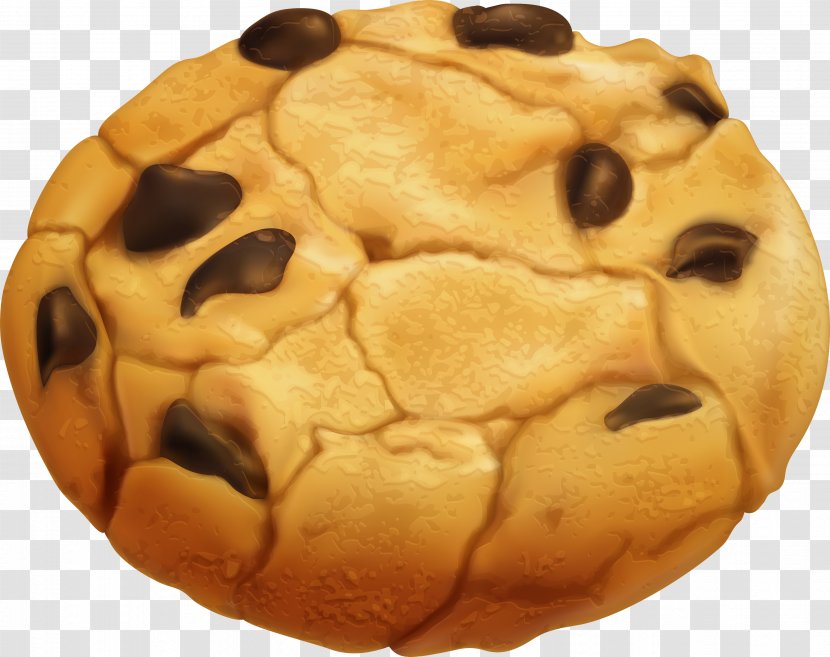This is an illustration of a round, nicely browned chocolate chip cookie placed on a gray and white checkered background. The cookie, depicted in a light brown hue with slightly darker brown crevices and jagged grooves, prominently features around nine to eleven chocolate chips of various shapes and sizes. These dark brown chips are unevenly scattered, with a noticeable cluster towards the periphery and one chip positioned near the side. The cookie shows characteristic craggy lines and slight melting of the chips, adding to its realistic, baked appearance. The textured detail and the checkered background give a digital or clip-art-esque vibe to the image.